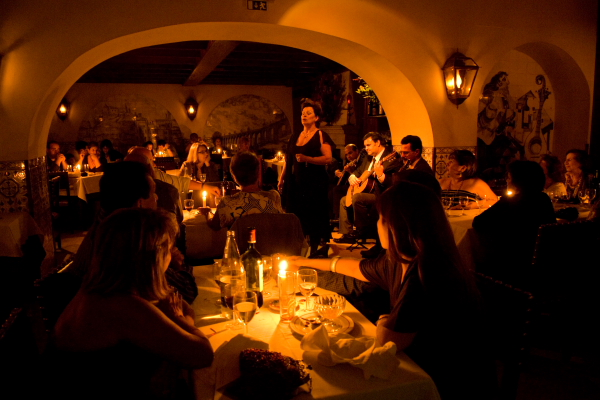In this intimate, dimly lit restaurant, a glowing atmosphere is created by candlelight and lanterns attached to the walls. The room, adorned with white tablecloths and wine glasses, is filled with patrons seated at various tables, all facing a small band providing live entertainment. Central to the scene is a woman in a black dress with short brown hair, standing beneath an archway on the right-hand side, passionately singing. Accompanying her, a man in a suit sits and plays an acoustic guitar, while another man, partially visible, likely plays a flute or harmonica. The back wall features two large circular designs flanked by lanterns, enhancing the cozy and elegant ambiance.